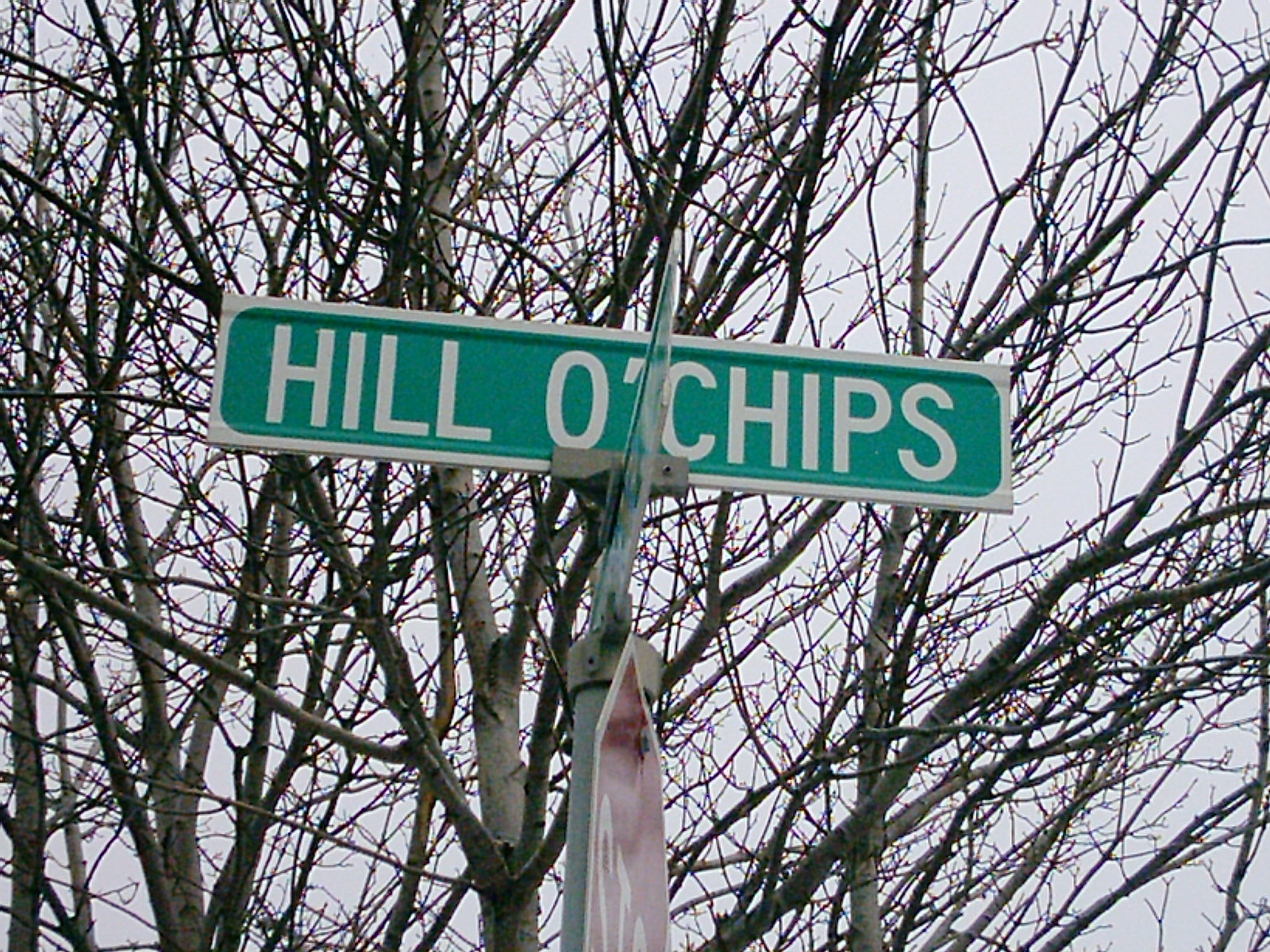In this photograph taken on an overcast day, viewers are positioned looking up at a street sign intersection. The main focus is the crossroad where the street signs and a stop sign meet. The upper street sign, green with a white border, prominently displays the name "Hill O' Chips" in white letters. Just below it, another street sign is attached but is turned perpendicular to the camera, making its lettering unreadable. A familiar red stop sign is partially visible below the intersection. Dominating the background are bare, leafless trees, their branches stark against the gray sky, suggesting it is either late fall or winter. The sky itself is uniformly bright gray, adding to the scene's bleak, wintry atmosphere.